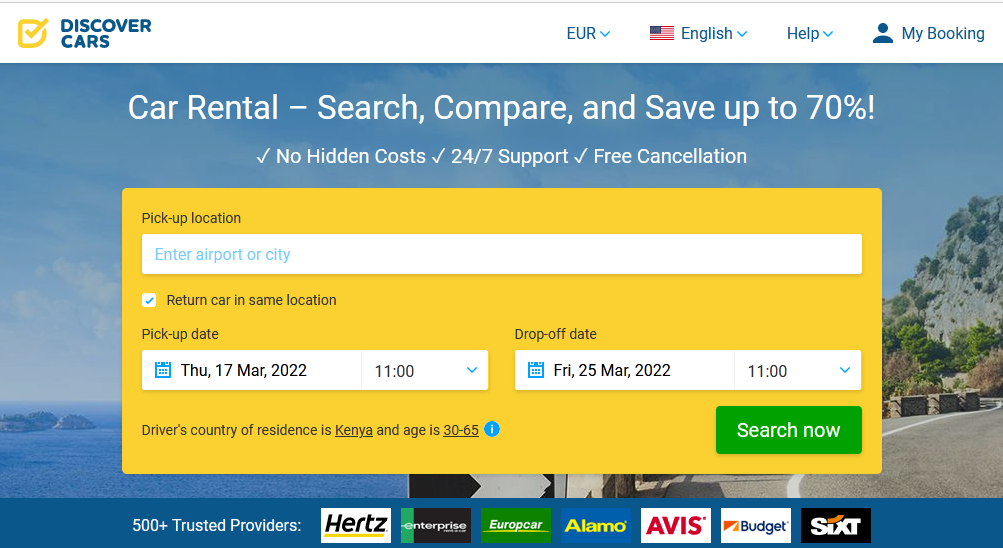The image is a screenshot from the Discover Cars website. At the top of the image, there is a white navigation bar featuring several elements. On the upper left corner, there is a yellow logo consisting of a letter "D" with a check mark inside it. To the right of the logo, the company name "Discover Cars" is displayed in blue text.

On the upper right side of the navigation bar, there are several options including a Euro currency symbol accompanied by a drop-down box, an "English" language option also with a corresponding drop-down box, and a "Help" option with a similar icon. Further to the right, there is a "My Booking" section with a user icon next to it.

The main section of the image prominently features a picturesque scene with a bright blue sky dotted with white clouds, an expanse of water, and a beach area on the right. Over this scenic background, text overlays highlight the website's offerings: "Car Rental - Search, Compare, and Save up to 70%," "No Hidden Costs," "24/7 Support," and "Free Cancellation."

Below the promotional text, there is a functional search box designed for users to input their pickup location and specify if they wish to return the car to the same location. Additionally, users can select their pickup and drop-off dates using the provided fields.